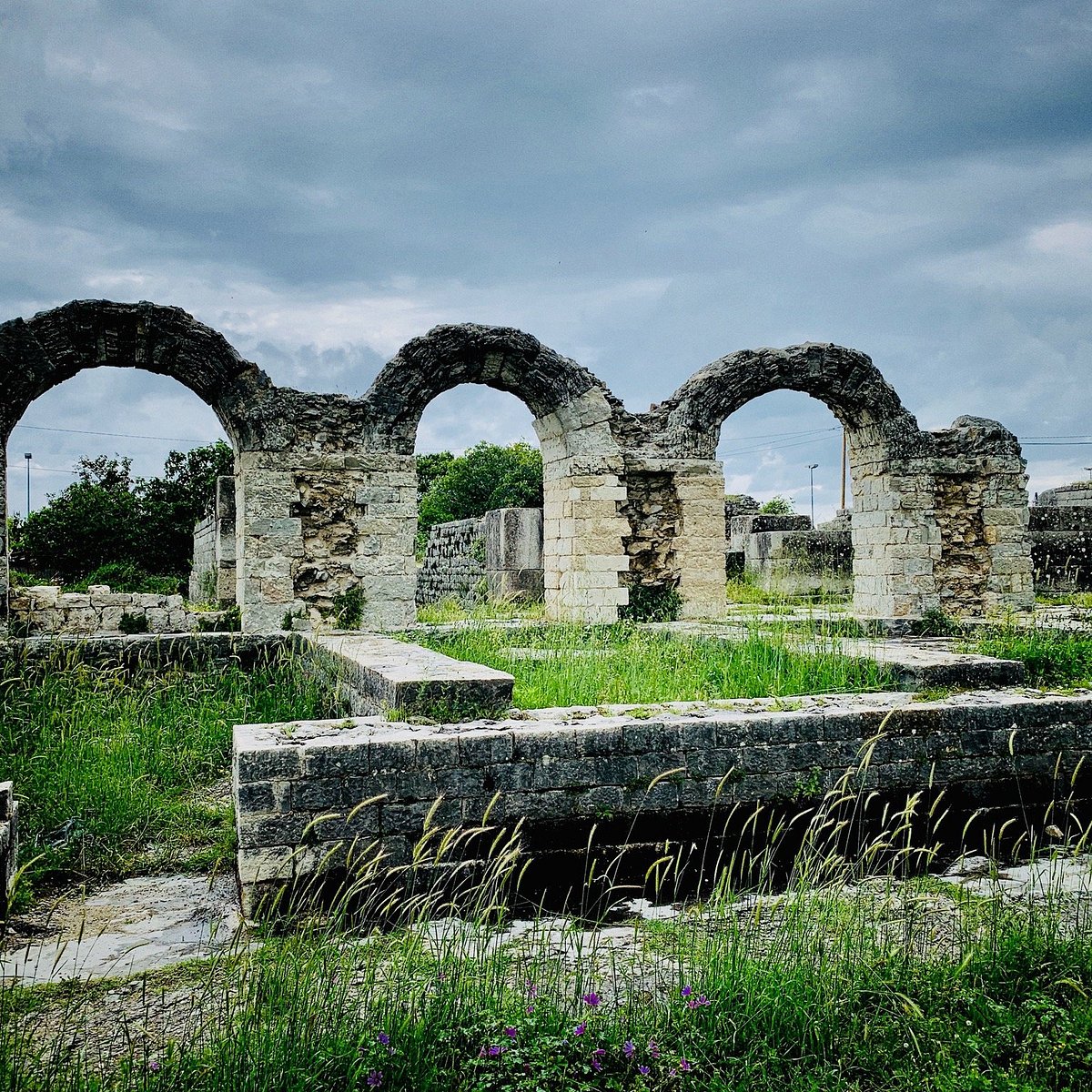The photograph captures an overgrown grassy field just outside a forest on an overcast day, with gray clouds blanketing the sky. Three stone arches resembling the McDonald's logo, made of eroded white stone, stand prominently in the center. These arches, remnants of an old architectural structure, are surrounded by foundations of small stone walls that segment the area. The grass, standing about four inches high, and various weeds indicate neglect. Scattered bricks and large stone pieces suggest the remains of a once-standing building now succumbing to natural decay. Behind the arches, additional stone walls can be seen, extending in various directions, with treetops rising beyond them. On the left side of the image, power lines and a streetlight near the trees are also visible, adding to the scene's historical juxtaposition.